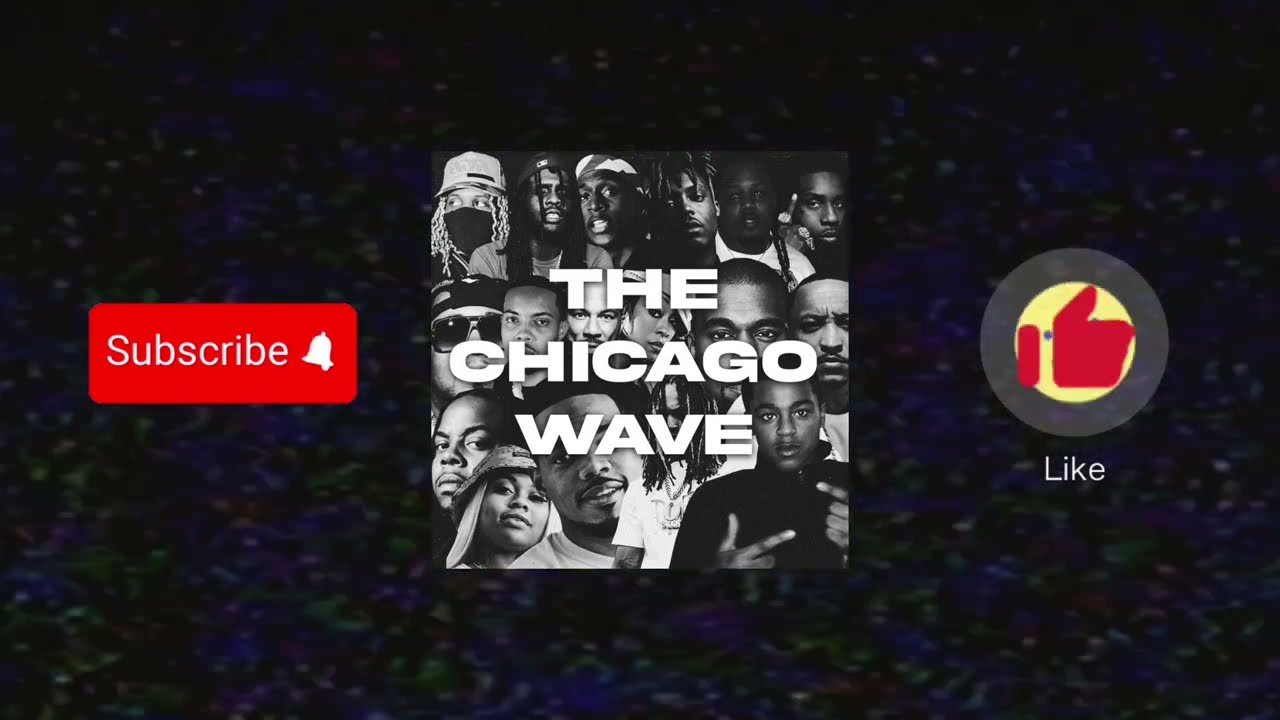This image features a central black and white square filled with faces of numerous people in three rows, displaying a variety of expressions such as smiling, frowning, and one person wearing a COVID mask. In the center of this square, bold white capital letters spell out "THE CHICAGO WAVE." To the left of this square, there is a red rectangular icon with the word "SUBSCRIBE" in white letters and a white bell notification icon beside it. On the right side, there is a circular icon containing a red thumbs-up symbol, encircled by a yellow ring, and the word "LIKE" written in white underneath. The entire backdrop of the image consists of a gradient of green and blue dots set against a black background.